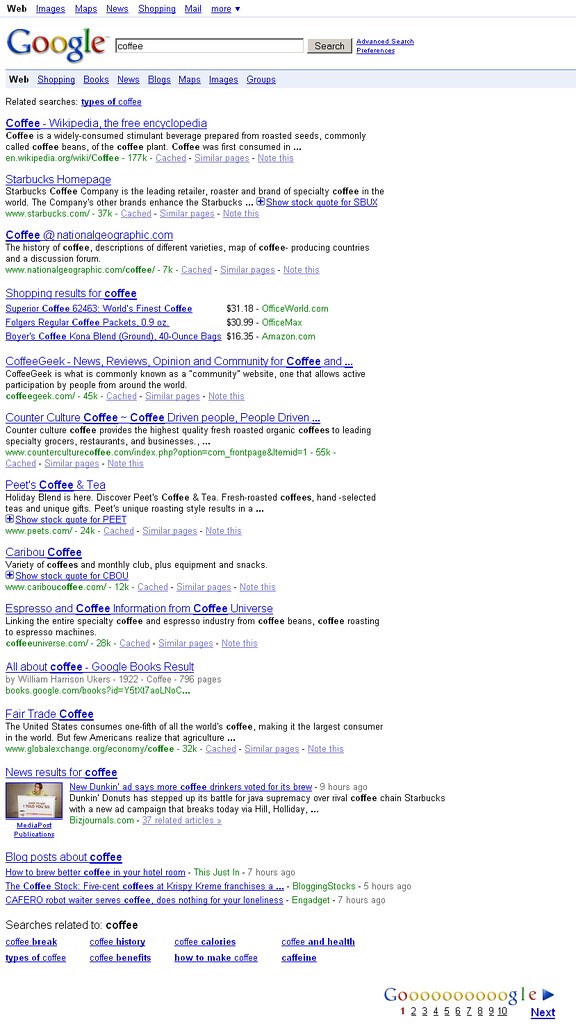This image depicts a screenshot of a Google search results page. In the upper left corner, the word "web" is prominently displayed, followed by options for "links," "images," "maps," "news," "shopping," and "mail" towards the right. Beneath these options lies the iconic "Google" logo with a search bar to its right, featuring the search query "coffee" and a search button adjacent to it.

Below the search bar, under the section titled "Related Searches," is the suggestion "types of coffee." The search results begin with:

1. **Wikipedia entry:** 
   - Title: *Coffee - Wikipedia, the free encyclopedia*
   - Description: "Coffee is a widely consumed stimulant beverage prepared from roasted seeds, commonly called coffee beans, of a coffee plant."
   - URL: `wikipedia.org/wiki/coffee`

2. **Starbucks Homepage:**
   - Description: "Starbucks Coffee Company is the leading retailer, roaster, and brand of specialty coffee in the world. The company's other brands enhance the Starbucks..."
   - Highlighted link: `Starbucks`

3. **National Geographic Coffee Page:**
   - Title: *Coffee at nationalgeographic.com*
   
Following these main search results, a section for shopping results for coffee products is displayed, including:
- Superior Coffee 62463
- World’s Finest Coffee, priced at $31.18, available at `officeworld.com`

This detailed capture provides a comprehensive overview of the prominent links and information presented in a typical Google search for "coffee."